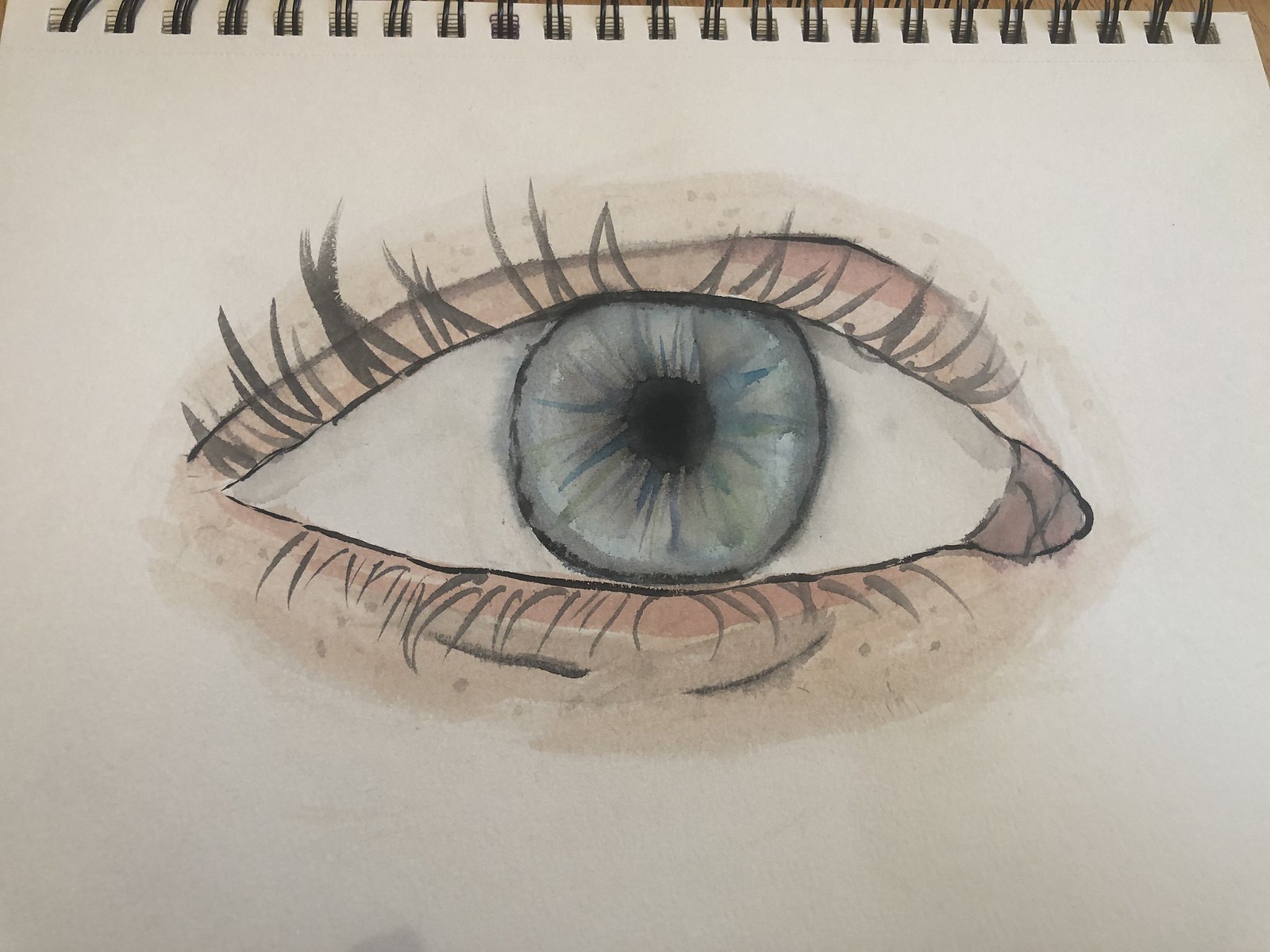This detailed watercolor illustration captures a close-up of a human right eye, centrally framed on a piece of paper in a spiral sketchbook, visible from the metal rings at the top. The iris displays a striking grayish-blue color with hints of green and brown, encircling a stark black pupil. The sclera is meticulously rendered in pure white, devoid of red veins, emphasizing the eye's clarity. The eye is adorned with long, dark brown or black eyelashes that fan out elegantly from each corner. Surrounding the eye are pale, peachy skin tones, indicative of Caucasian skin, with additional darker peach shadowing on the eyelid for depth. Notably, a small tear duct is precisely illustrated, and a few freckles are scattered underneath the eye, adding to the realism. The attention to detail and nuanced color work highlight the artist's skill in creating a lifelike depiction.